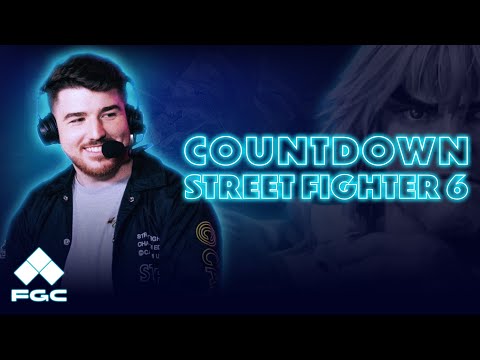This advertisement poster, formatted in a horizontal rectangle with thick black borders at the top and bottom, features a prominent depiction of a young, attractive Caucasian man with medium-length black hair and a pleasant smile. He wears headphones with a microphone extending to his mouth and is dressed in a black jacket adorned with gold patches and white snaps over a gray or possibly white t-shirt. The man is cut off at the stomach level by the bottom black border. To the right of him, the bold text "Countdown" appears in large black letters with a neon blue outline, followed by "Street Fighter VI" in similar stylings just below it. Over his right side, a triangular monogram with three squares and the letters "FGC" in white can be seen. A slightly visible, blurred image of a woman with blonde, scraggly hair and large eyes appears faintly in the upper right corner, her face partially obscured by the text. The background behind her features a bluish-green hue, giving the overall image a vibrant yet intense look, befitting the theme of the "Street Fighter VI" game.